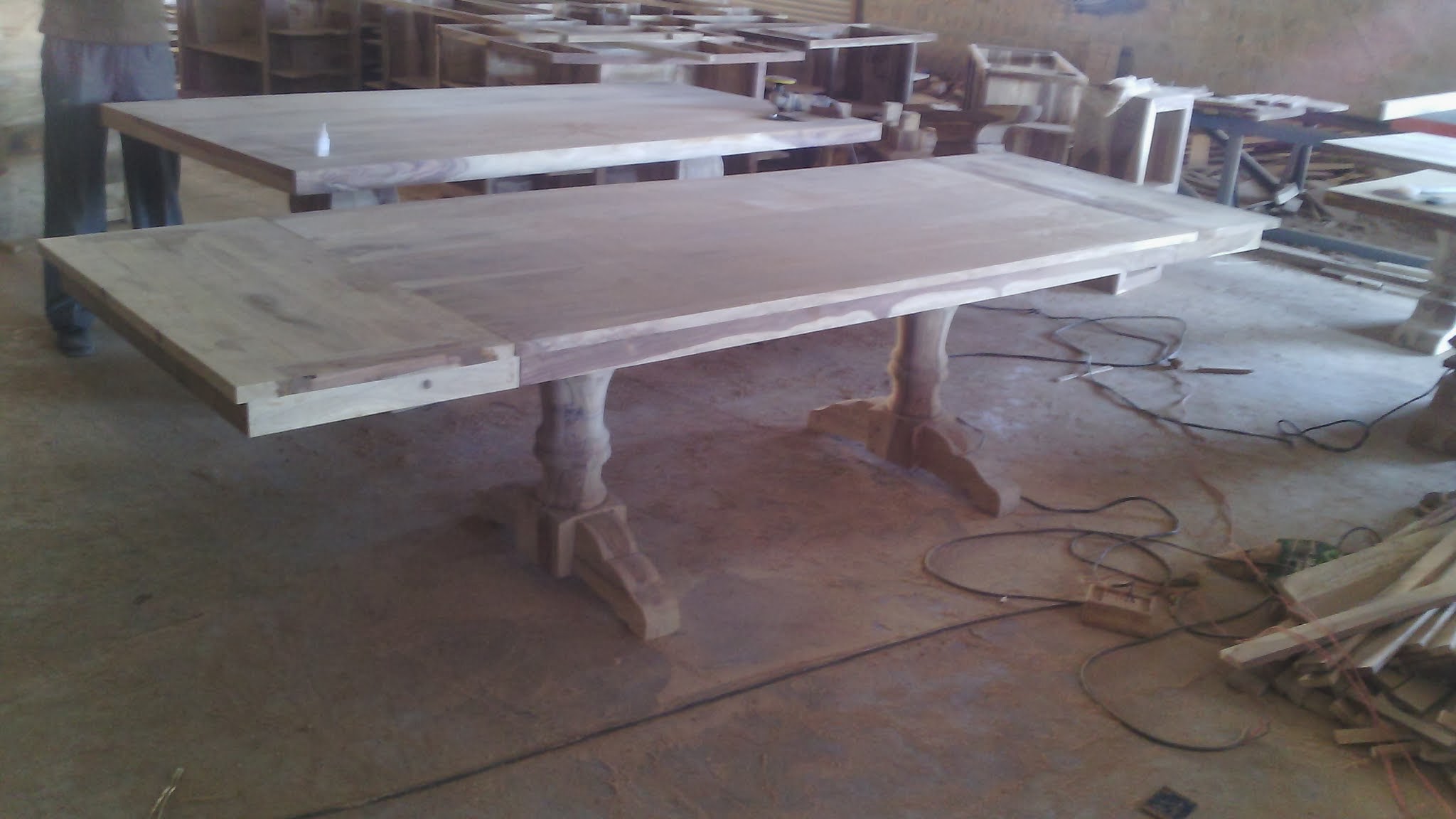The image captures a detailed scene inside a large warehouse dedicated to carpentry work. The floor appears to be composed of multiple concrete slabs, with scattered wiring and lengths of wood. In the foreground, there is a large, unfinished wooden table with ornate T-shaped legs, yet to be varnished. Just behind it is a smaller table, both showcasing fine woodworking craftsmanship. The far wall is lined with various pieces of furniture and frameworks in different stages of completion. The top right corner of the image shows more smaller wooden tables. Amidst the setup, in the top left corner, a man is partially visible from the waist down, wearing grey pants and presumably a brown or olive green T-shirt, or possibly a brown apron. The scene is vibrant with the organized chaos typical of an active woodworking area.